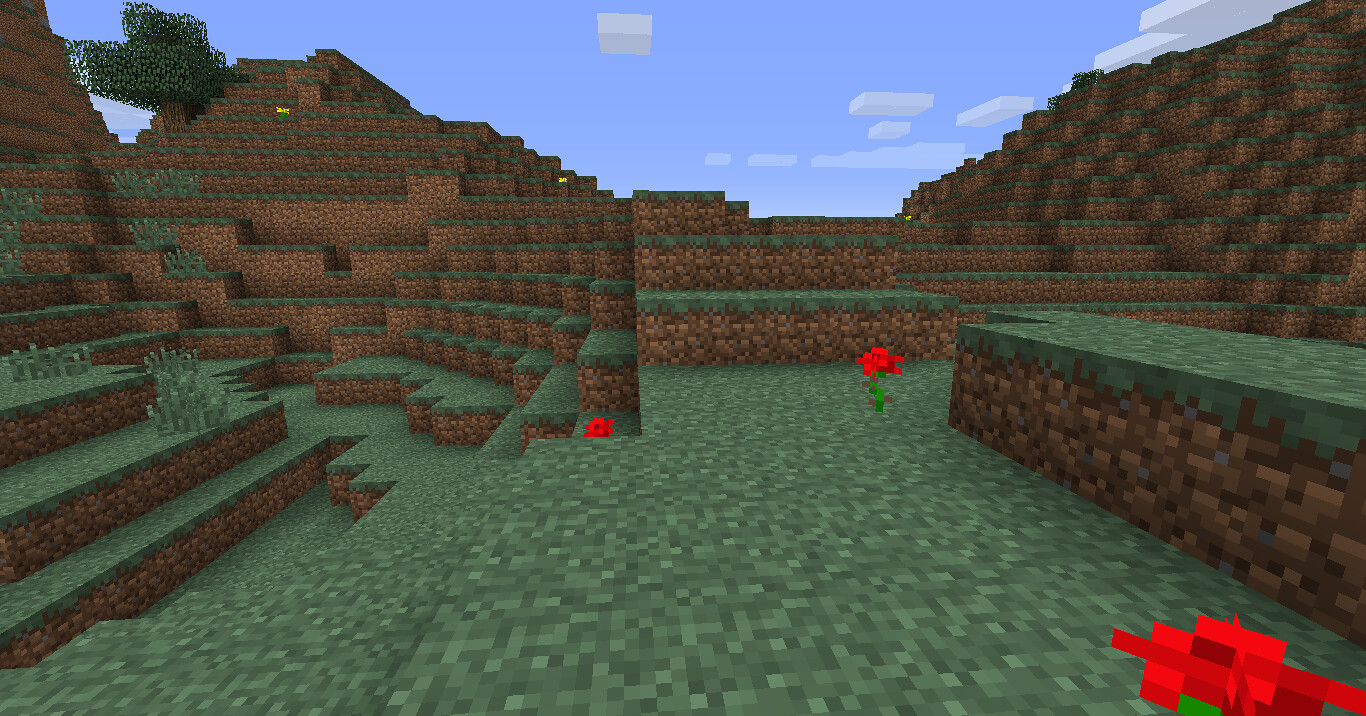This is a screenshot from the popular video game Minecraft, characterized by its distinctive, pixelated graphics and cube-shaped blocks. The scene is set in a terrain featuring numerous hills and mountains, primarily composed of dirt blocks topped with dark green, splotchy grass that varies in shades from light to medium to dark green. The environment is dotted with bright red flowers and, in the distance on the left side, patches of grass and a few yellow flowers come into view. A tree is also visible in the upper left corner. The sky forms a vivid blue backdrop, adorned with several fluffy, cube-shaped clouds, completing the iconic Minecraft landscape.